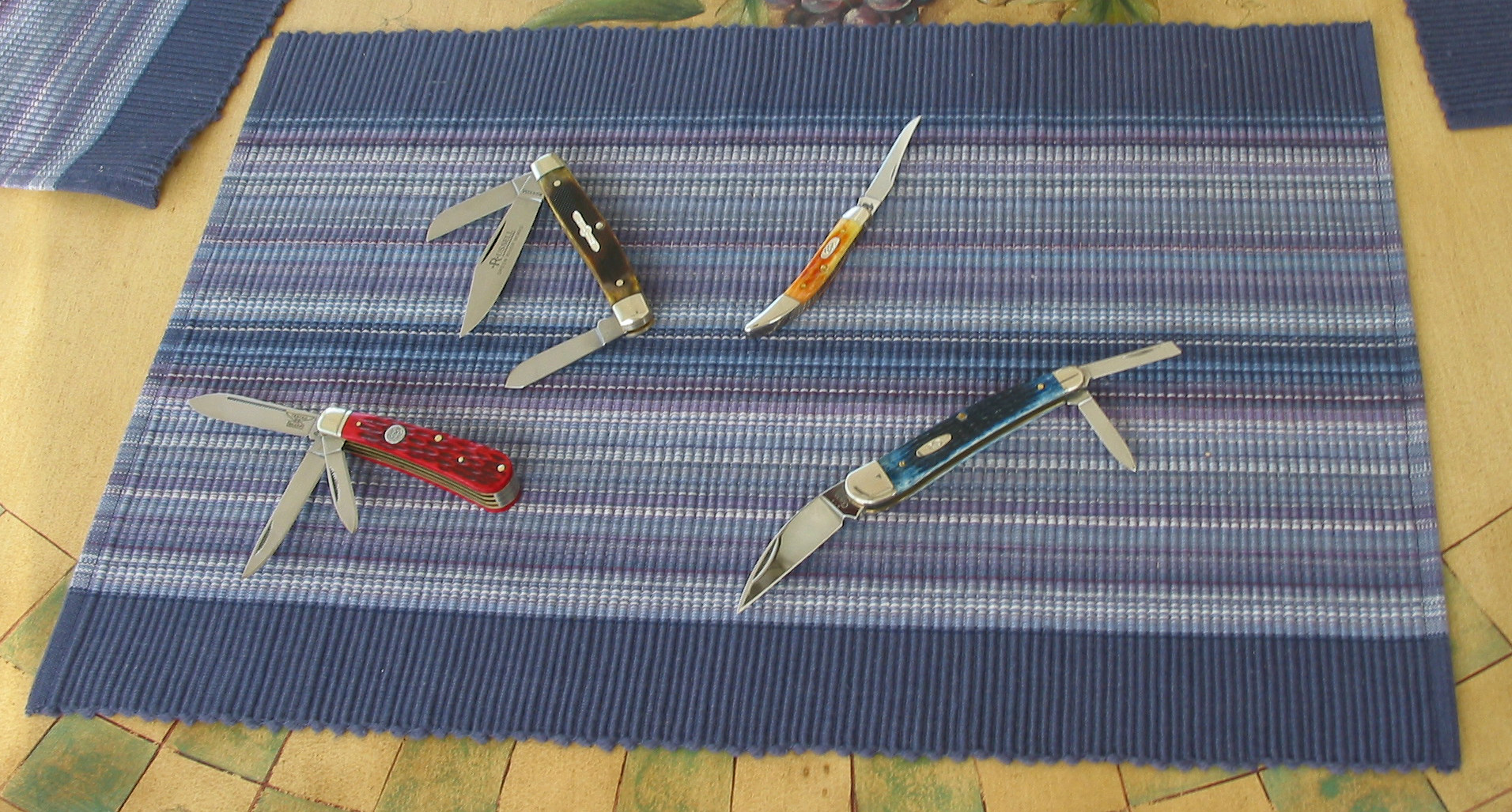The image depicts a collection of four small pocket knives arranged on a blue and purple striped placemat, which is set on a flat surface indoors. The knives are meticulously displayed with all their blades open. From left to right, the first knife has a dark red handle and features three blades extending from the top. The second knife, with a yellowish-brown handle, has two blades coming out of the top and one from the bottom. Next is an orange-yellow knife, noticeably thinner than the others, with a single blade extending from the top. The final knife has a deep blue handle with two blades on one side and a larger blade on the opposite side. Each handle appears to be made of bone with stained colors, adding a unique character to each knife. The placemat serves a dual purpose of enhancing the visual presentation and protecting the knives from scratches or damage.